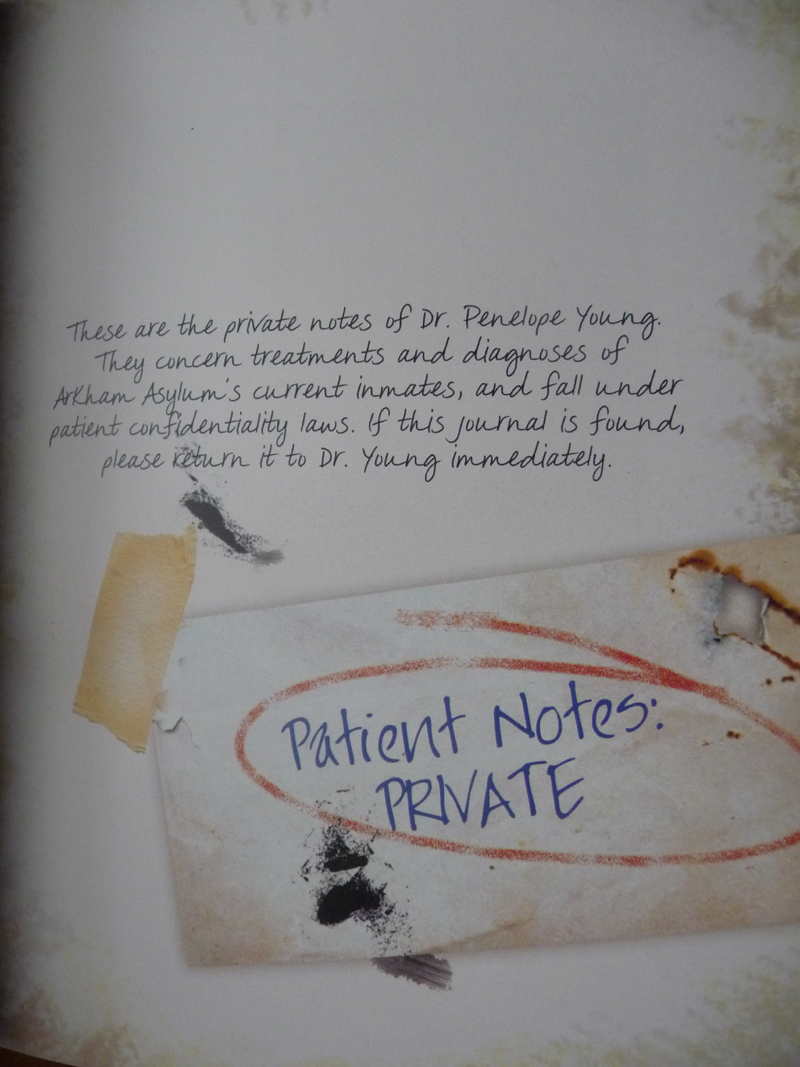The image appears to be a digitally created collage, possibly from a computer or graphic program. It depicts what looks like a piece of paper taped to another piece, with a realistic appearance of the tape. The outer edges of the image are slightly blurred, adding to the digital nature of the collage. The main content consists of a document with a handwritten-style script that reads: "These are the private notes of Dr. Penelope Young. They concern treatments and diagnoses of Arkham Asylum's current inmates and fall under patient confidentiality laws. If this journal is found, please return it to Dr. Young immediately." Below this text, there is an additional piece of paper taped onto the document, and within a red oval circle are the words "patient notes, private" written in blue ink. The document also features smudges and fingerprints, adding to its realistic yet possibly virtual appearance, suggesting it may be part of a computer game.